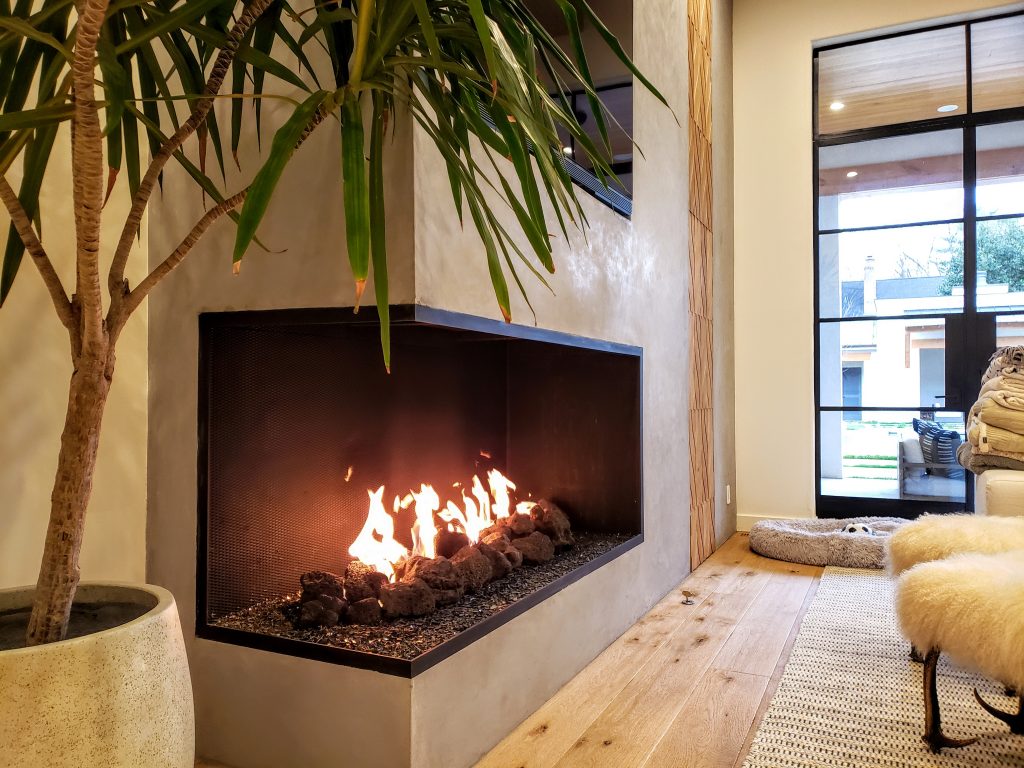This detailed image captures an elegant fireplace set within a luxurious residential space. The tan-colored wall houses a built-in fireplace, which features a black trim and realistic-looking faux logs ablaze over decorative rocks. A significant architectural detail is a rectangular cut-out that protrudes from the wall, housing the sleek, modern fireplace. Positioned in front of this cozy fireplace is a furry beige couch and a plush rug that spans over light wooden floors, adding warmth to the room's ambiance. To the side, a sophisticated floor plant, possibly a palm or a fern, stands tall in a smooth, round white planter, enhancing the room's opulent decor. A nearby dog bed with a soccer ball lies in waiting, adding a touch of homey comfort. Footstools or low chairs with wooden legs and fluffy beige tops are partially visible, further enhancing the cozy atmosphere. Large windows in the background flood the space with natural light, hinting at an expansive view of the outside world. This inviting scene suggests an ideal lounge area perfect for relaxation.